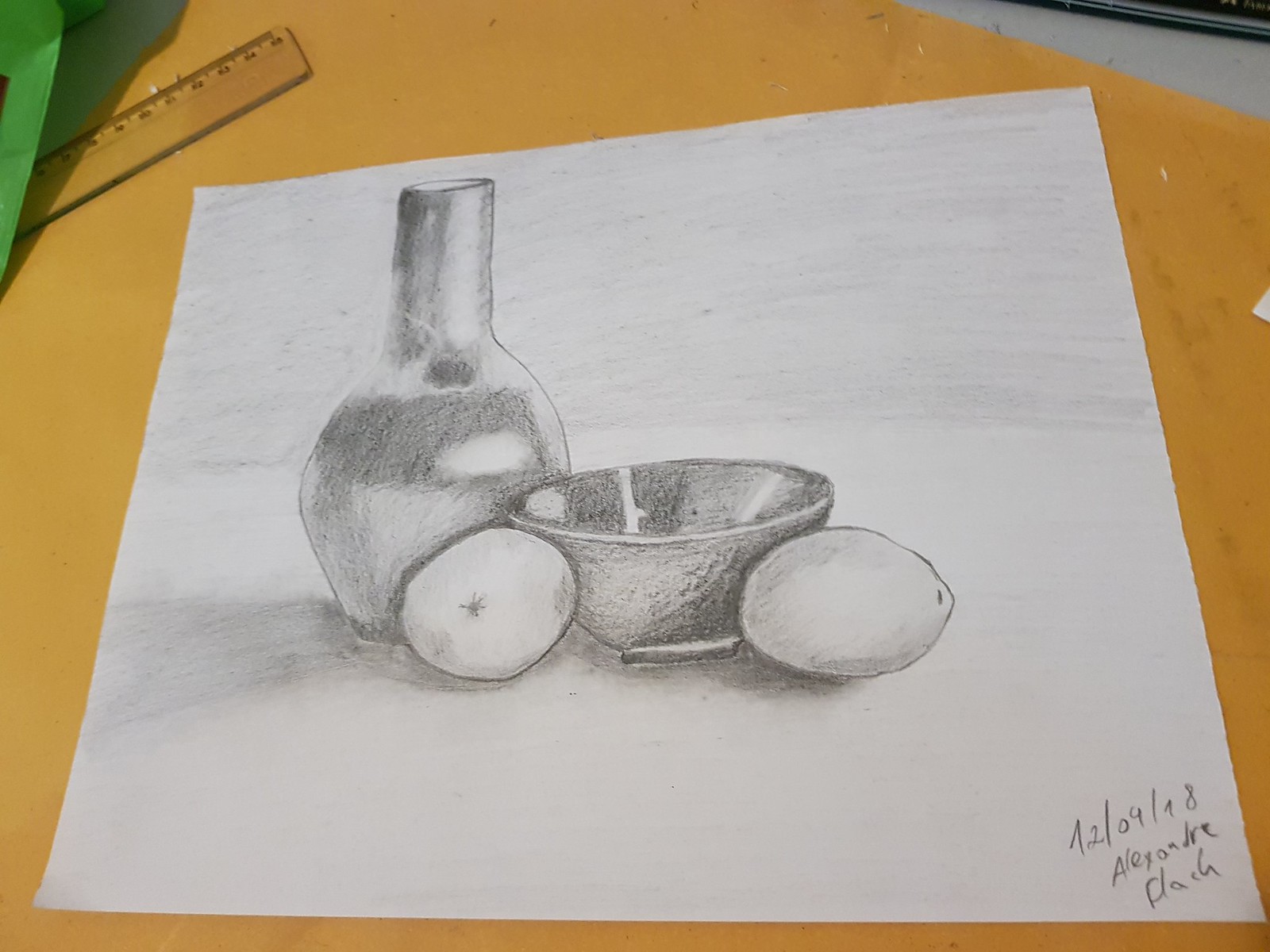A detailed still life sketch, primarily in pencil or charcoal, depicted on a smooth, large, white piece of paper placed against a primarily yellow background. The top left corner of the image reveals a tan and black wooden school ruler. An additional part of a translucent ruler protrudes near the top edge. The sketch features a vase (or ewer) on the upper left with lighter shading and a bulbous shape tapering into a narrow neck. To the right of the vase, at the center, is a darker gray stoneware bowl. In front of these objects are two rounded fruits, possibly lemons, apples, or potatoes, positioned on either side of the bowl. The bottom right corner of the drawing is signed "Alexandre Floch," with the date "12-09-18." There is also a faint indication of a green bag towards the left side of the image. Additional subtle shadows and a light gray background hint at depth and dimension in the composition.